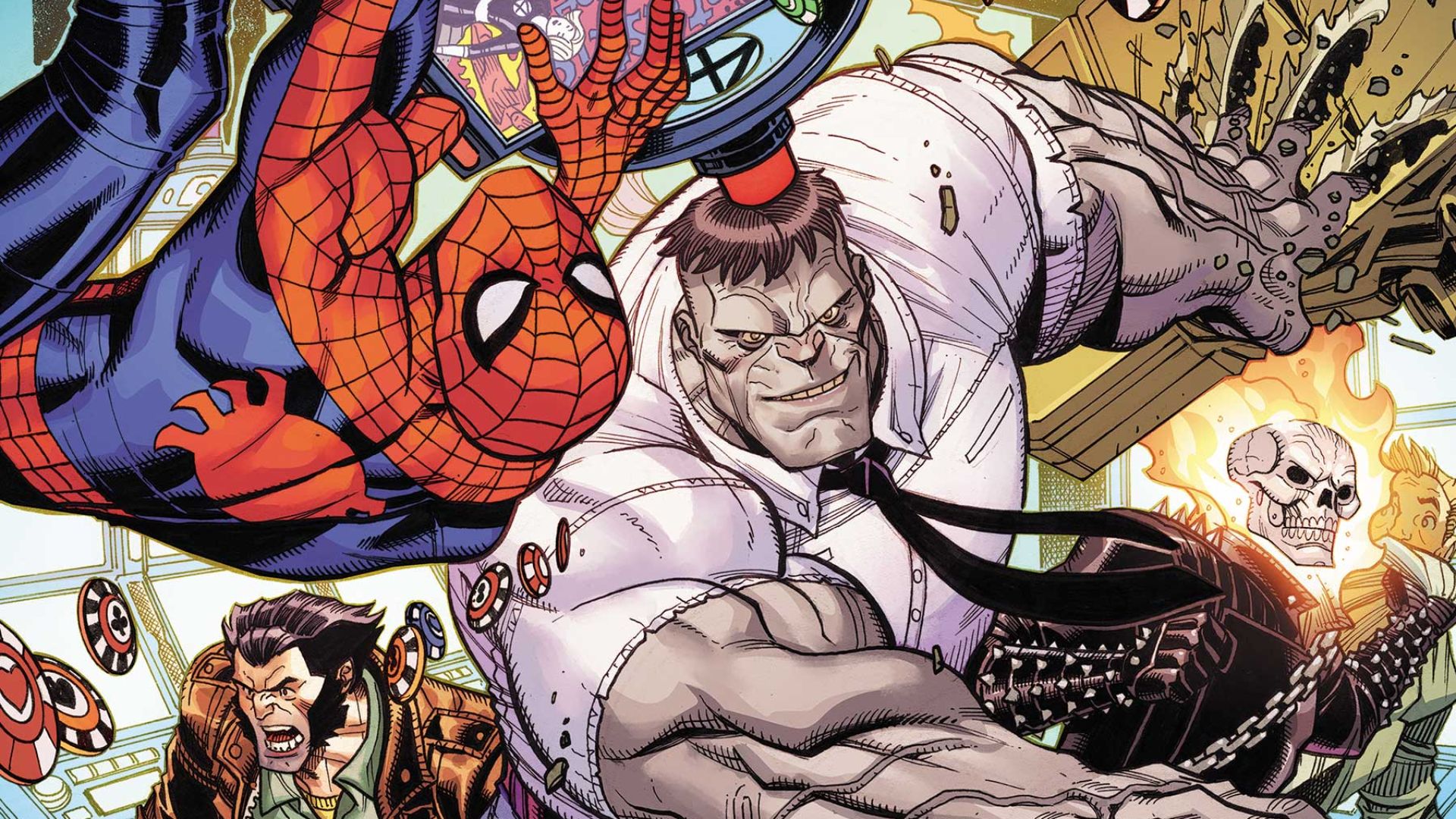In this horizontally rectangular, full-color cartoon image, several superhero characters are dynamically depicted in a chaotic scene. Dominating the center is an enormous, gray-skinned man with incredible muscles, slanted eyes, and a square jaw. He's wearing a very small hat on his head and a short-sleeved white shirt with a tie. This character resembles a gray version of the Incredible Hulk, though uniquely dressed. His left hand, with serrated edges on his fingers, appears to be pulling up a bridge, while his right hand is out of the frame but hinted to be connected to chains.

To the left of this giant figure, Spider-Man can be seen prominently in his red and blue costume, hanging upside down as if climbing a glass section of a building with windows visible beneath him. Below Spider-Man, another fierce-looking superhero with long brown hair, a beard, and a brown jacket—likely Wolverine—is poised and ready for action. He exudes a menacing presence with his muscular build and fierce expression.

On the right side of the gray giant, a flaming skull with a gold boundary around it, identified as Ghost Rider, adds to the tumultuous scene. His leather jacket and chains are also visible, contributing to the sense of impending conflict. The image is also scattered with casino playing chips flying around, adding an additional layer of chaos and intrigue to the otherwise intense superhero confrontation.